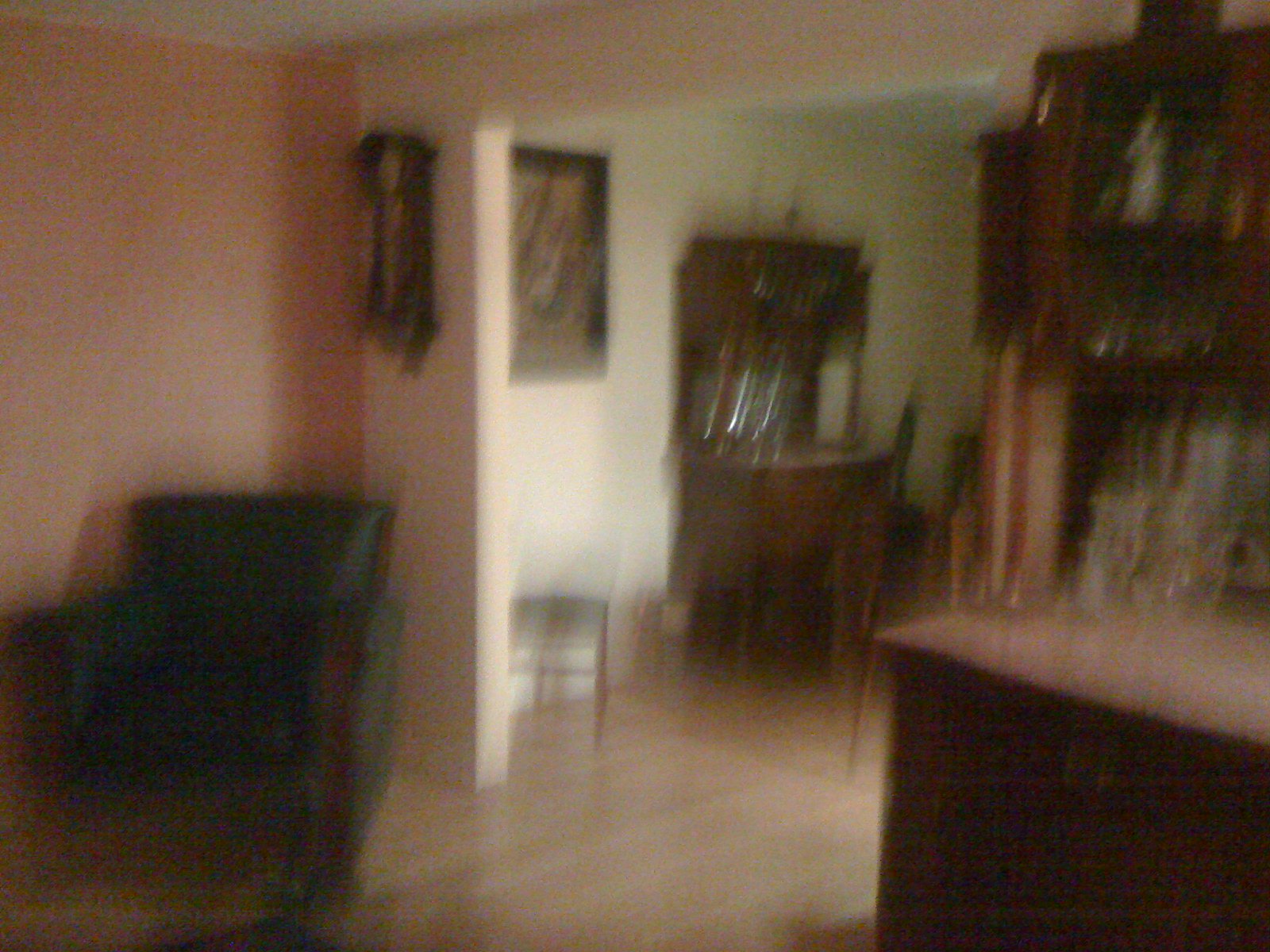This blurry photograph captures the interior of a home, likely taken from a den or living room looking into an adjacent room through a roughly six-foot wide doorway. In the immediate foreground, a black leather armchair or easy chair sits cozily in a corner beneath an old-fashioned, dark wood clock—possibly a cuckoo clock—mounted on a light brown or peach-colored wall. The armchair is against a small section of wall where the opening to the other room is visible. The floor of this area is light-colored hardwood.

In the adjacent room, there's an ornate, antique-looking piece of furniture, potentially a Hoosier or a hutch, featuring a dark wood finish and topped with a light surface that could either be marble or covered in white linen. This piece is adorned with various knick-knacks, including some crystals and possibly a couple of pitchers. Nearby, there's a smaller chair or stool. In addition, the adjacent room has light tan or off-white walls and another similar antique piece of furniture with glass cabinet doors, shelves, and what seems to be a mirror backing.

On the walls, both rooms feature traditional decorative elements, including framed wall art in dark frames. The kitchen area, visible in part, showcases dark wood cabinets contrasted by light countertops. Overall, the image, though blurry, hints at a traditionally styled, comfortably furnished home with a blend of antique and practical pieces.